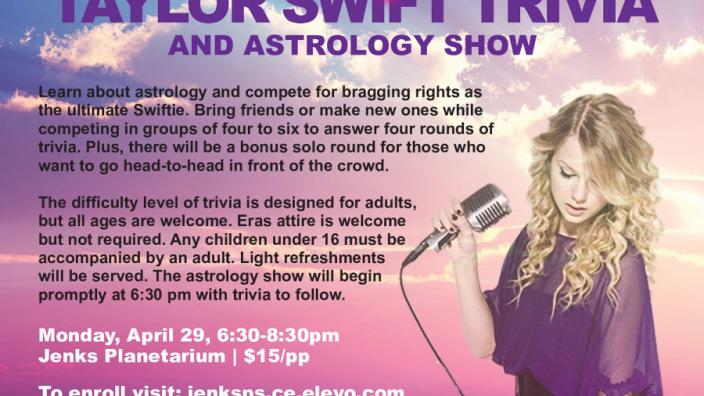This digital graphic features a promotional poster for the "Taylor Swift Trivia and Astrology Show." The background transitions from a blue and white sky at the top to a purplish hue, creating a twilight effect. At the top, large capital letters in purple read "Taylor Swift Trivia," and below it, "Astrology Show" is written in a smaller, sans-serif font.

On the left side of the poster, two paragraphs provide detailed information about the event. Here, attendees are invited to learn about astrology and compete for bragging rights as the ultimate "Swifty." Participants can join with friends or form new teams of four to six members to answer four rounds of trivia. There’s also a bonus solo round where individuals can go head-to-head in front of the crowd. While the difficulty level is tailored for adults, all ages are welcome.

To the right, there is an old photo of a teenage Taylor Swift. She has long blonde hair cascading towards her chest and is captured looking downward to the lower right. Taylor is donning a purple shirt with mesh shoulders and black pants while holding a classic, metallic silver microphone with a visible black cord.

At the bottom of this poster, in white text, the event details are listed: "Monday, April 29th, 6:30 to 8:30 p.m. Jenks Planetarium. $15 per person. To enroll, visit Jenks-CE.inLevo.com."